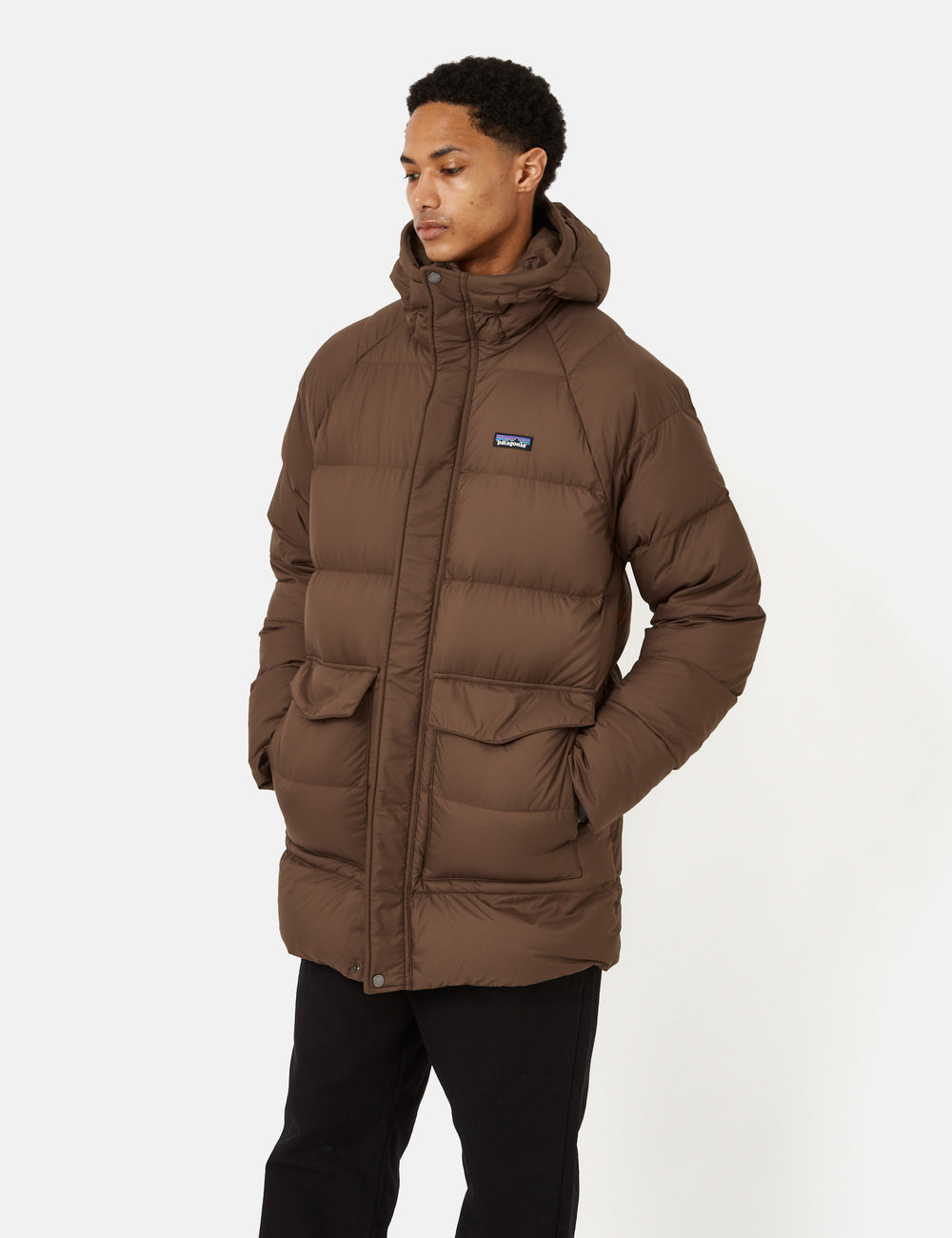The color photograph captures a young African-American male model in his 20s standing in front of a clean, white background. He is facing the camera at a slight angle, allowing for a full view of his front from the knees up. The model has short, curly brown hair and a composed expression, looking down slightly. He is showcasing a brown Patagonia puffer jacket, identifiable by the small, blue, white, and black logo on the left chest. The jacket features a hoodie, which is down, and extends up to just below his chin. There are two front pockets with flaps at the top, and beneath these, two additional side zipper pockets where the model has his hands tucked in. The brown puffer jacket also has buttons running from just below the chin to the bottom of the coat. Completing his look, the model wears black pants, accentuating the jacket's design. The photograph's clarity highlights the model and clothing in a bright and well-lit setting, devoid of any other objects or text, ensuring the focus remains solely on the attire.